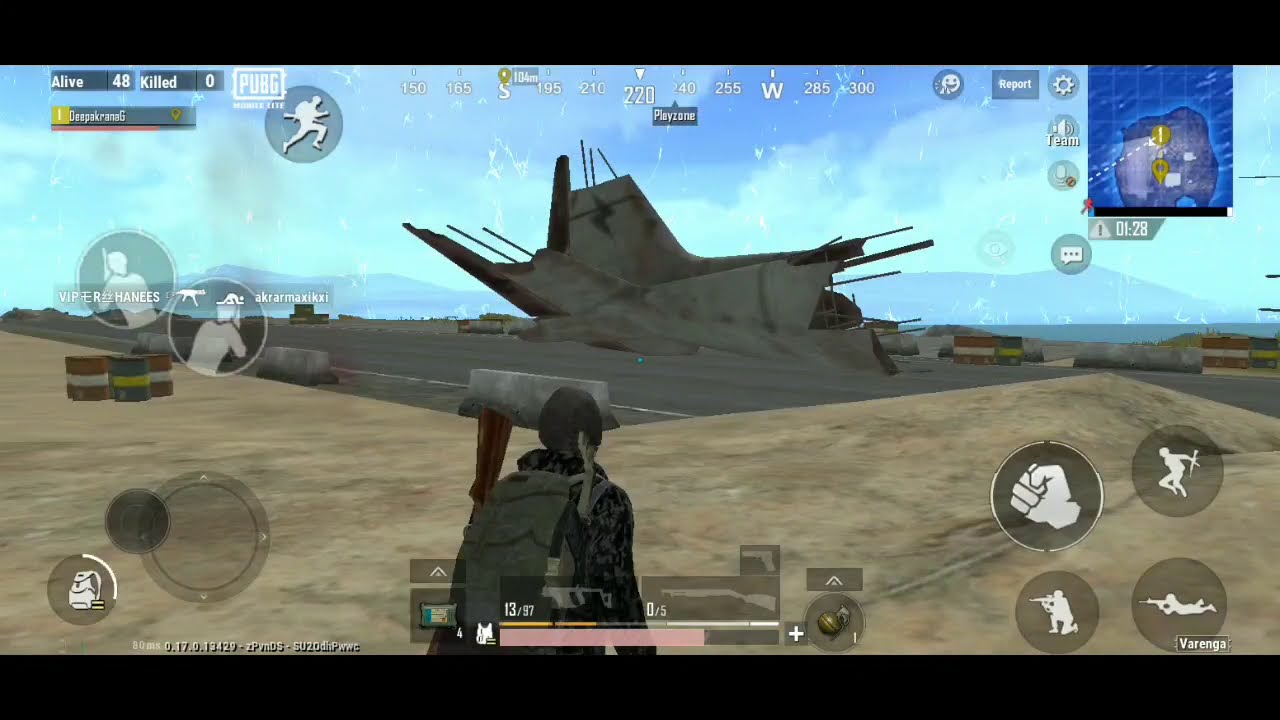The image depicts a detailed screenshot from the mobile game PUBG (PlayerUnknown's Battlegrounds). The background features a clear blue sky with a silver and brownish structure that appears to be a building or bunker, possibly resembling a crashed airplane. This structure is set against a backdrop of a dirt field and an asphalt strip. The foreground shows the player character, seen from behind, standing about four feet from the camera's elevated perspective. The character wears a long-sleeved black and gray shirt, a gray backpack, and possibly a hat or helmet. A rifle is visibly attached to the side of their backpack, with the butt extending above their left shoulder.

The heads-up display (HUD) is rich with information, spanning the edges of the screen. The top left corner reads "alive 48, killed 0", indicating the player's current status, alongside the PUBG logo and a run icon. The top right corner displays a map, highlighting an island in dark blue amidst blue water. The bottom center of the screen features a health bar, weapon choices, a grenade, healing items, and commands for different actions such as punch, jump, crouch, and lay down. The bottom left corner includes a movement joystick icon and a backpack icon, with lean left and right shortcuts above. The bottom right corner shows additional stances the character can assume, including crouched and prone positions, depicted by corresponding icons of a person with a gun.